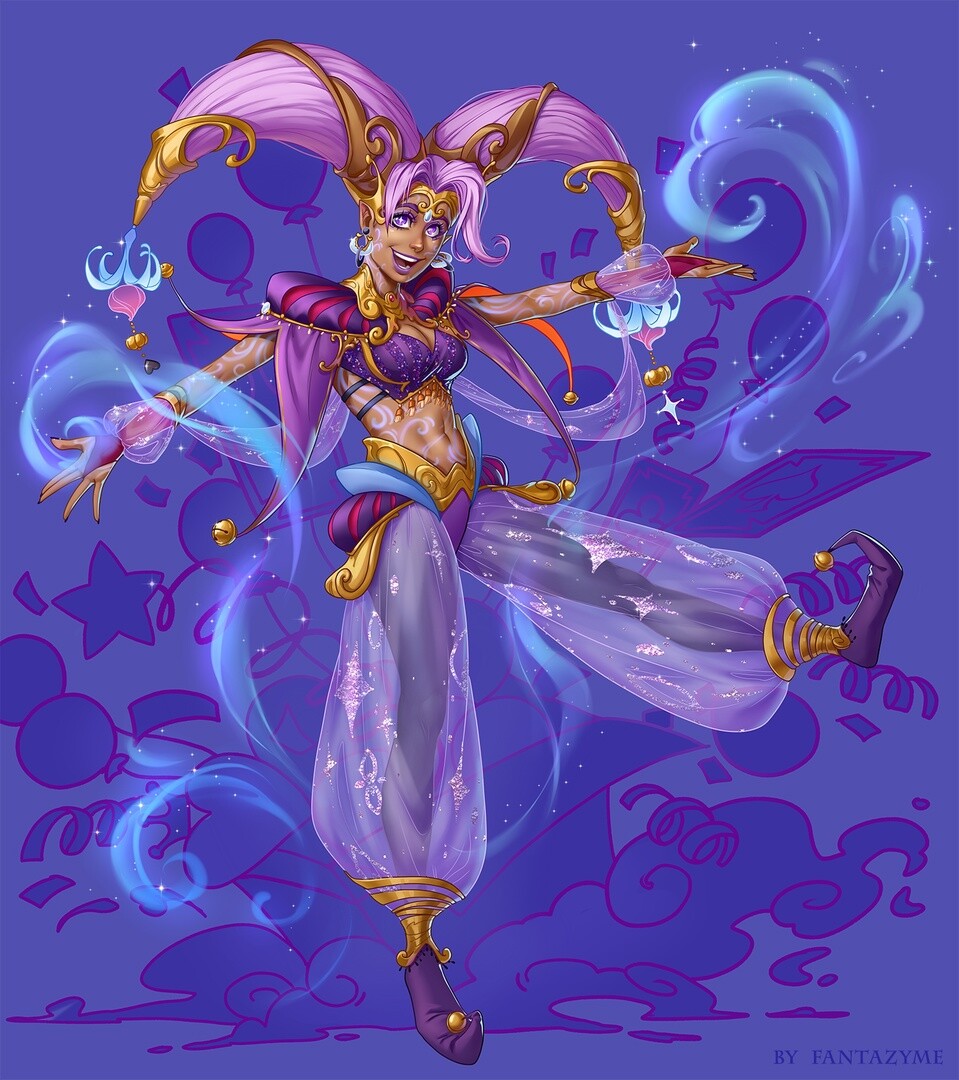The artwork by Fantazine, located in the lower right corner, depicts a vibrant, Aladdin-inspired female figure. The character is designed with striking details, including a highly ornate and ostentatious headdress. Her appearance draws immediate attention with her lively dance pose, smiling expression, and arms gracefully extended. She wears a jewel-adorned purple bikini top that reveals her belly button and a pair of see-through, fluffy purple genie-style harem pants, cinched with a gold ring at the bottom. The character’s ensemble includes maroon gloves with gold trim and elf-like shoes that curl up at the toes, each adorned with a bell.

She has distinctive light purplish-pink hair styled into voluminous pigtails with intricate swirls framing her face, and she is adorned with abundant jewelry. Her makeup includes striking purple eyeshadow and lipstick, complementing her white hoops and purple eyes. Her skin is embellished with delicate light purple swirly designs.

The backdrop of the image is a magical night sky colored in various shades of purple, featuring a playful array of confetti, balloons, stars, and whimsical doodles like open boxes, cars with playing card symbols, and streamer-like lines. This artistic creation exudes a festive and enchanting atmosphere, capturing the essence of a whimsical genie-like dancer in a fantastical setting.